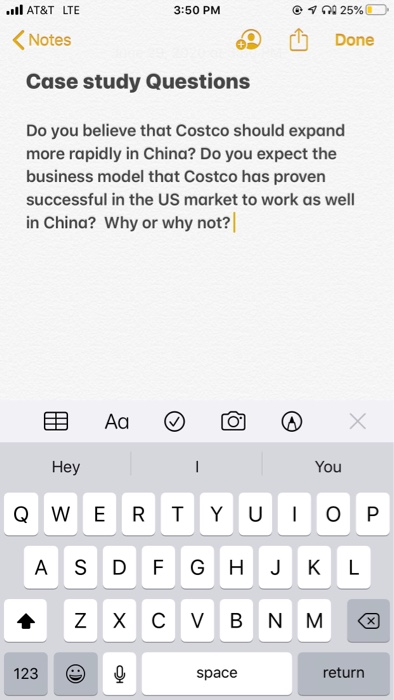This image is a screenshot of an Apple device's Notes application, captured in portrait orientation. The device is connected to the AT&T network, as indicated by the logo and LTE symbol in the upper left corner, with the current time displayed as 3:50 p.m. The status bar also shows cell signal strength and a battery level at 25% in the upper right corner.

At the top of the Notes app, the title "Notes" appears in the upper left corner accompanied by a left-facing caret icon, suggesting a navigation option. On the right, there is a "Done" button and two additional icons.

The content of the note is titled "case study questions" and contains the following text: 

"Do you believe that Costco should expand more rapidly in China? Do you expect the business model that Costco has proven successful in the U.S. market to work as well in China? Why or why not? China is becoming more and more consumer capitalist in its society."

At the bottom of the screen, the Notes app icons are visible, and the on-screen keyboard is displayed for text input. The yellow cursor is positioned at the end of the phrase "Why or why not?" indicating the person has just typed this note. The context suggests that the individual is preparing case study questions, likely for a class, seminar, or policy discussion.